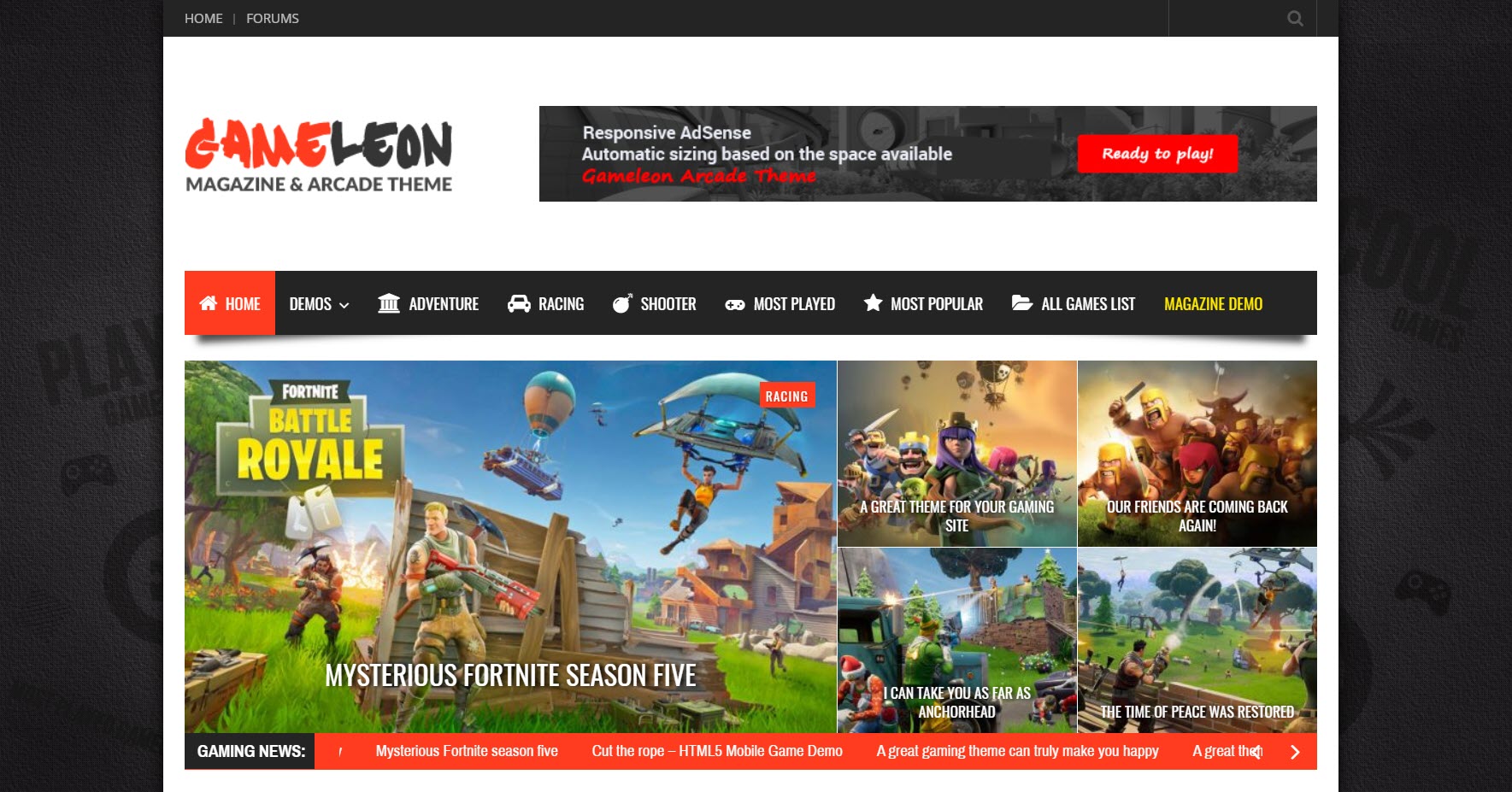This screenshot captures the homepage of a gaming website named "Game Leon," which features a distinct red and black color scheme. The logo, placed at the top left, displays "Game" in red and "Leon" in black, with a tagline below that reads "Magazine and Arcade Theme" in black text.

The website layout includes various articles and advertisements for popular games. The most prominent feature is a large article at the bottom left about "Fortnite Battle Royale," showcasing an image of players using gliders and engaging in colorful combat. The accompanying white text reads, "Mysterious Fortnite Season 5."

On the right side of the screen, four smaller articles are arranged in a grid format:

- The top left article includes the headline: "A Great Theme for Your Gaming Day."
- The top right article, which appears to discuss "Clash of Clans," carries the headline: "Our Friends Are Coming Back Again."
- The bottom right article is another "Fortnite" piece, titled "That Time and Place Was Restored."
- The bottom left article seems somewhat incomplete but mentions, "I Can Take You As Far As you... As Far As Anchorea." 

Overall, the website features vibrant game-related content designed to attract and engage avid gamers.